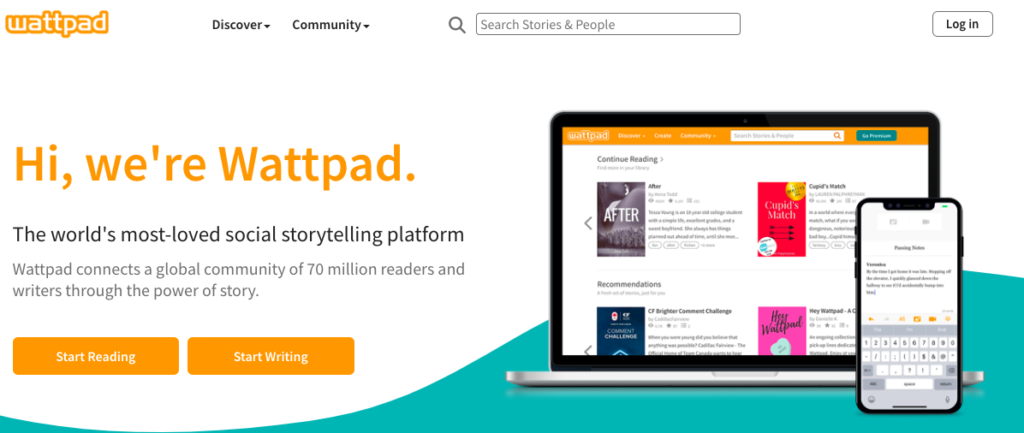Advertisement for Wattpad Platform: Showcasing the leading social storytelling platform, this promotional image spotlights Wattpad's widespread appeal. At the top, bold text reads "Wattpad" alongside key terms "Discover" and "Community." Below is a search bar labeled "Search stories and people" and a login icon. The central message proclaims, "Hi, we are Wattpad, the world's most loved social storytelling platform. Wattpad connects a global community to 70 million readers and writers through the power of story. Start reading, start writing." 

To the side, a computer display showcases popular books, including titles from the 'After' series, while a smartphone alongside it displays various written works, emphasizing the platform's accessibility across devices. This visually engaging image captures Wattpad's essence, inviting users to explore a world of stories and join a vast, interactive community of readers and writers.